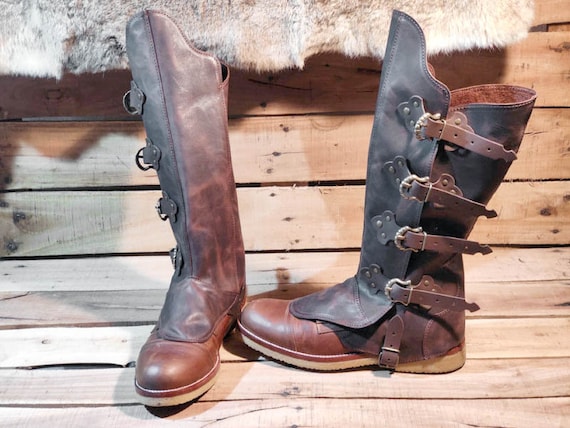The photograph captures a pair of dark brown leather boots resting on an old, unfinished wooden bench. The bench, composed of what appear to be light pine planks, extends both as the base and backdrop of the image. Draped over the top of the bench is what looks like a piece of cowhide or fur. Positioned in an L shape, one boot is facing forward with the toe pointed towards the camera, while the other boot is oriented to the side. These boots are detailed with classic-looking buckles, having four on each boot along the shaft and an additional clasp on the lower part. The boots seem to be well-used but maintain a clean appearance, suggesting they might be rugged riding boots often associated with cowboy attire. The soles of the boots are visibly lighter and made of white rubber, providing a subtle contrast to the rich, dark leather.